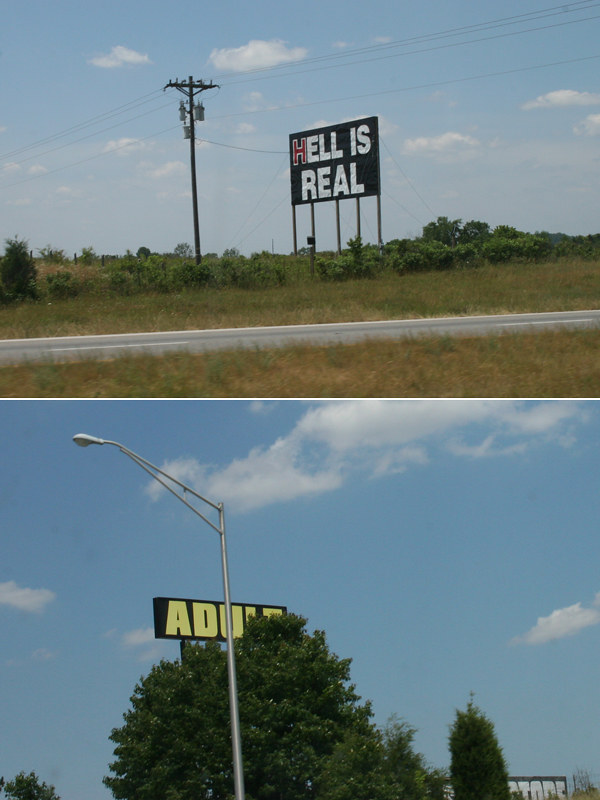The image is a collage of two separate photographs stacked vertically with a small white space dividing them. The top photograph features a small, narrow road flanked by grass on each side, extending into the distance where a brown telephone pole and electrical wires can be seen. Dominating the upper part of this image is a rectangular billboard with a black background that reads "H ELL IS REAL" in bold white letters, with the 'H' notably in red. The sky above is light blue with scattered, small white clouds, indicative of a bright daytime scene.

The lower photograph showcases a tall silver streetlight standing in front of a green-leaved tree. Partly obscured by the tree and streetlight, there is a black billboard with the word "ADULT" written in yellow, though only the letters "ADU" are clearly visible due to the obstruction. In the bottom right corner of the billboard, "STORE" is written in white lettering. This image also captures a similar sky, light blue with white clouds, consistent with the time of day portrayed in the first photograph.